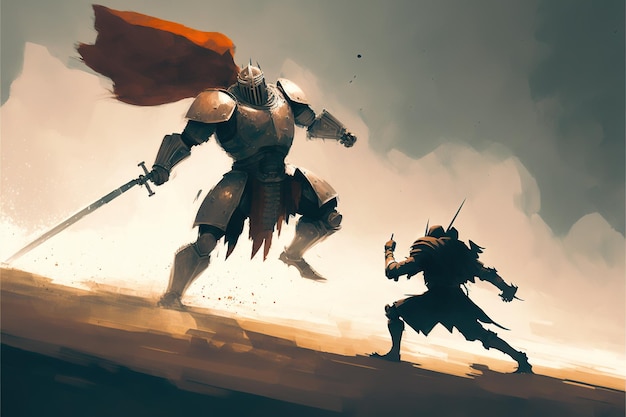The image portrays a dynamic, fantasy-themed digital painting of an exhilarating battle scene between two warriors. The larger combatant, on the left, stands atop a dusty hill, projecting an imposing figure about eight or nine feet tall. Clad in traditional European-style armor, he is covered from head to toe in metal plates, with pronounced shoulder pads, a slitted-visored helmet, gauntlets, and armored boots. His striking red cape billows behind him as he holds an enormous, intricately hilted sword in his right hand, positioned to deliver a mid-jump, descending attack. To the right, the smaller, agile fighter appears silhouetted and backlit, his features obscured but his essence clear. Wearing more flexible leather armor with some metal components for added protection, he wields a small knife and carries additional weapons, including a bow strapped to his back, suggesting a versatile combat style. The electrifying scene is set on a sloped, sandy terrain with dust particles suspended in the air, emphasizing the movement and intensity of the moment. The backlighting further adds to the cinematic quality, creating an engaging, energetic fantasy illustration reminiscent of a fervent battle poster.